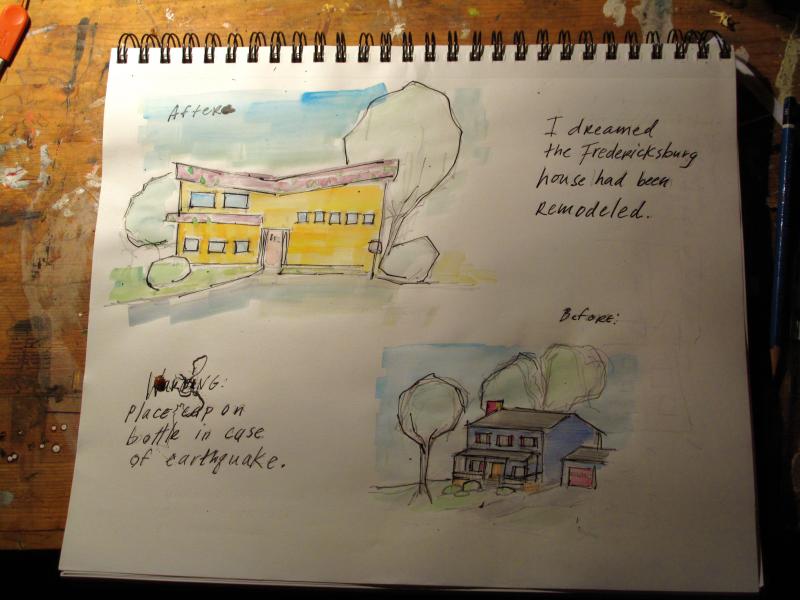This image captures a sketchbook, identifiable by its multiple sheets of paper bound together by metal rings at the top. The sketchbook is open to a page featuring architectural drawings, specifically depicting a house in two stages: before and after a remodeling. The before drawing illustrates a spacious blue, two-story house with a peaked gray roof, a red chimney, and a blue garage with a gray roof and red door. The surroundings include green trees, bright green grass, and bushes under a clear, blue sky.

The after drawing presents a remodeled version of the house, now yellow in color with a uniquely sloping "V" shaped red roof. The remodeled house appears to maintain its multi-story structure and features a red door, accompanied by trees and bushes in the landscape.

Above the drawings, the text reads, "I dream the Fredericksburg house has been remodeled," highlighting the conceptual nature of the sketches. Below the illustrations, a note reads, "place upon bottle in case of earthquake," adding a whimsical or illustrative touch to the artwork. The drawings seem to be rendered in watercolor.

The sketchbook rests on a heavily-used drawing desk or drafting table, characterized by numerous paint and ink splatters. This detail contributes to the creative and dynamic atmosphere of the workspace.